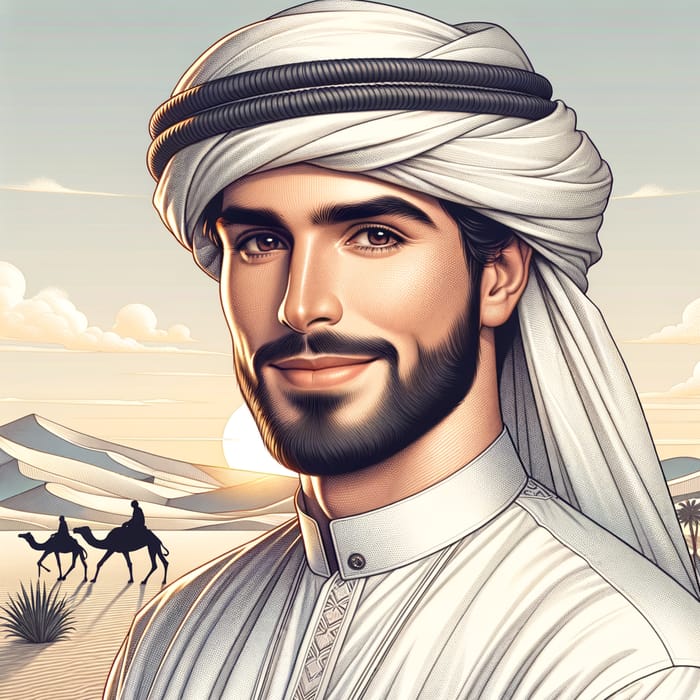This digital illustration captures a handsome Sheik, possibly a princely figure, portrayed from the chest up with a smile directed at the viewer. The Sheik, fair-skinned with a neatly groomed black beard and brown eyes, wears a traditional Saudi outfit consisting of a white shirt with a narrow mandarin collar adorned with a small button and a vertical stripe down the center. His head is covered with a pristine white turban, accented by two black bands.

The background depicts a desert landscape at sunset, with shades of golden yellow and orange painting the sky. Sand dunes and a large sand mound dominate the left side, while to the right, a tropical tree adds contrast to the arid setting. Silhouettes of two people riding camels appear to the left, their shadows cast long by the setting sun. The sandy terrain stretches out, creating a sense of vastness, and the sky above is dotted with clouds, enhancing the depth and realism of the scene. The combination of these elements creates a vivid and detailed portrayal that blends simplicity with an air of regality.